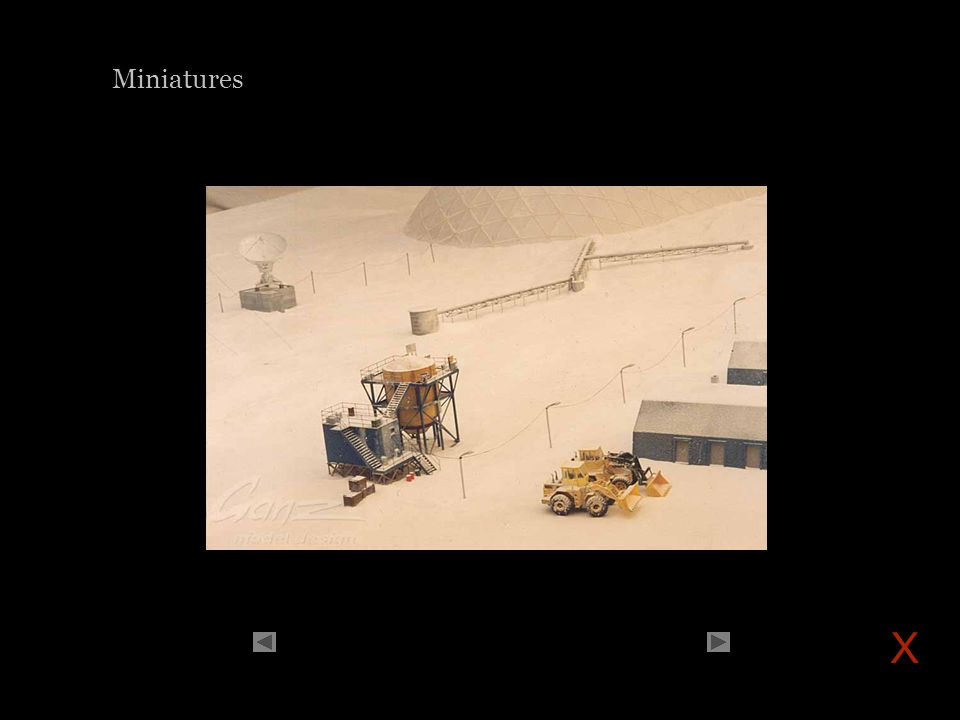The image displays what appears to be a screenshot featuring a detailed miniature model of an Arctic or South Pole base. The entire image is bordered by a thick black frame. In the top left corner, the word "Miniatures" is prominently displayed in white text. Dominating the center of the image, the scene depicts a snowy landscape populated with various structures and equipment: 

- Two earth-moving machines in the foreground, depicted in colors such as yellow and gray.
- A cylindrical water tank with a staircase leading up to it, positioned next to a small blue shack.
- Several blue and gray buildings and metal structures scattered throughout the scene.
- A geodesic dome and a dish antenna, resembling those used in deep-space communications, located on the left side.
- Overhead wires, possibly for lighting, stretching across the scene with shacks situated beneath them.

The setting is enhanced with additional details such as fences and a satellite dish near the top left, emphasizing the intricate nature of the miniature model. At the bottom of the screen, there are left and right arrows for navigation, and a red 'X' icon is situated in the bottom right corner, suggesting that this image was taken from a computer interface. The color palette includes shades of white, black, tan, brown, yellow, red, and gray.